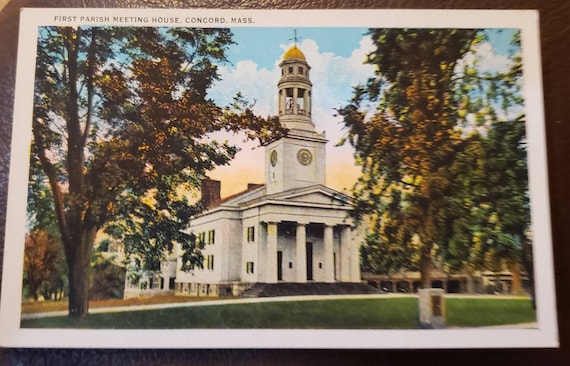The image is a vintage postcard showcasing the First Parish Meeting House in Concord, Massachusetts. Dominating the center is a grand white church with four to five prominent pillars at its entrance. Above the church rises a striking tower topped with a golden dome. The building also features several windows and black doors, with chimney structures visible on the left side. It is set against a backdrop of a clear, sunny sky with a few clouds, enveloped by lush greenery. Several trees flank the building, with a few having leaves turning color, hinting at the onset of fall. The foreground displays a well-kept grassy area, enhancing the natural, serene ambiance. The image has a slightly muted and aged appearance, suggesting it was taken many decades ago, focusing primarily on the majestic architecture of the church.